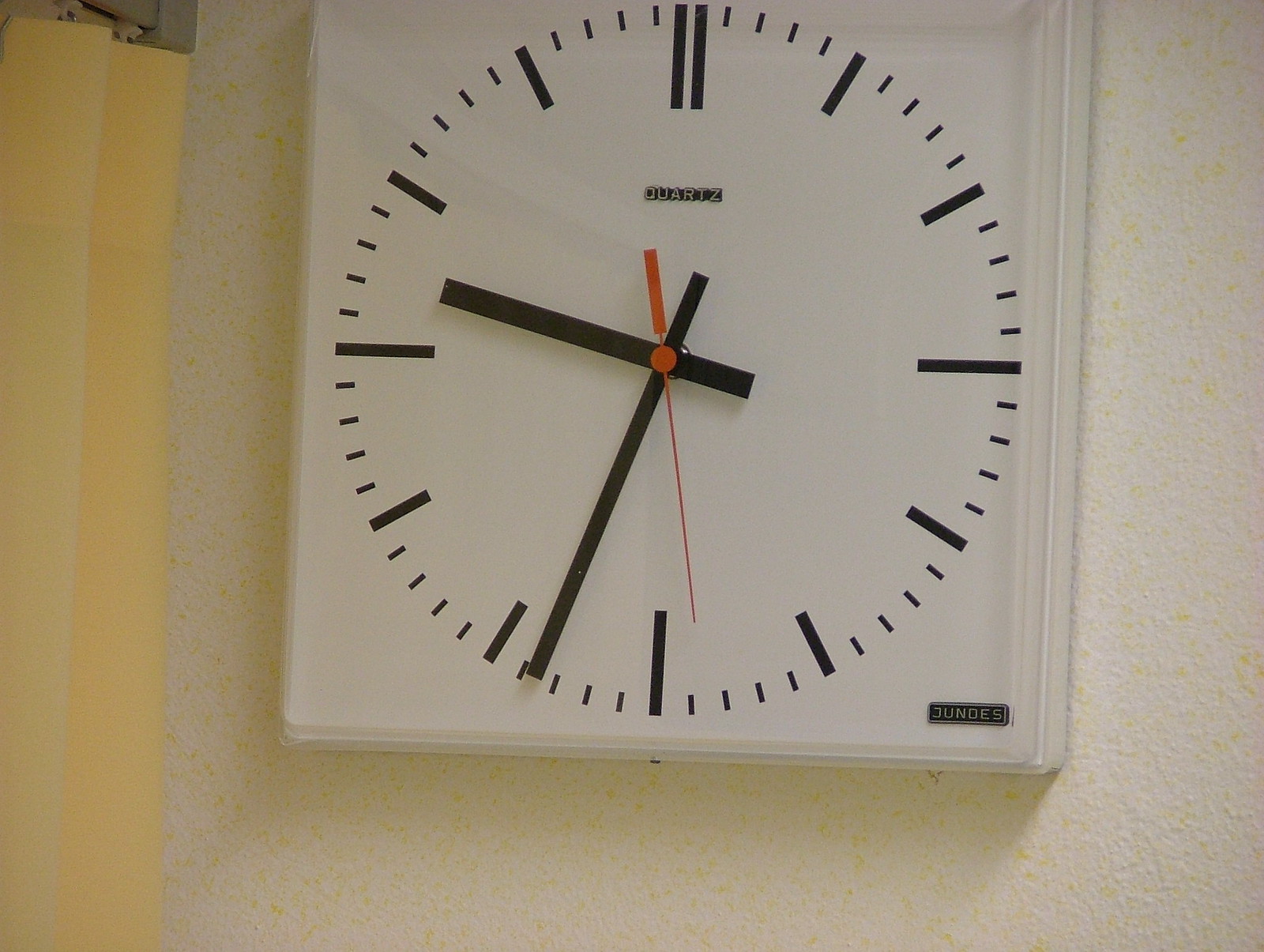This photograph captures a square white wall clock prominently displayed on an off-white wall, which features faint yellow flecks and a slightly bumpy texture. The clock, which has a white frame, shows a simple yet precise design: it lacks traditional numbers, instead using lines of varying lengths to mark the time. Two bold black lines denote the 12 o'clock position, a single bold black line indicates 6 o'clock, and thinner black lines mark the five-minute intervals. Even smaller black lines delineate each minute. The clock's face is round within its square frame, and it is home to three hands: the long black hour and minute hands, and a needle-shaped red second hand pointing at the 29-second mark. Directly below the 12 o'clock position is the word "quartz," set in a small black rectangle with white text. In the lower right corner, the label "JUNDES" is visible. The time displayed on the clock is 9:34. A portion of a yellow curtain can be seen on the right side, suggesting the clock is positioned near a corner.